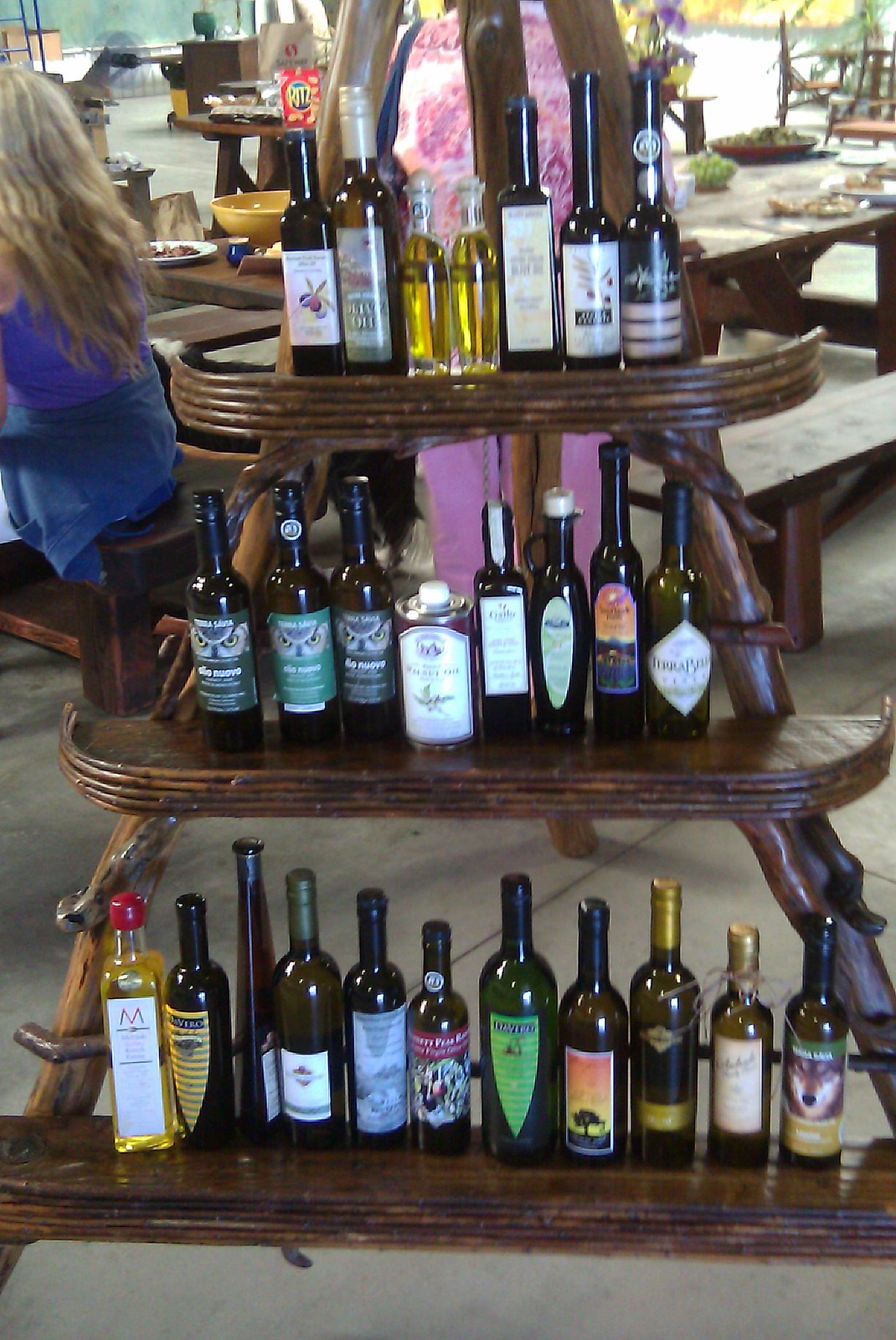The photograph captures a tiered display of shelves in a pyramid stack, each shelf narrower than the one below, all crafted from dark brown wood that might be olive wood, supported by a knotted wood-style triangular base resembling tripod branches. The shelves are adorned with an assortment of bottles, resembling wine or olive oil containers, with various distinctive shapes and sizes. The clear bottles reveal a yellowish liquid, suggesting they likely contain olive oil, given the branding and logos which include images of a wolf, an owl's eyes, and olive leaves, and names like Bavaro or Pavaro. Surrounding this main display, the background shows dark brown wooden benches and tables laden with different foods, plates, and a box of Ritz crackers. A woman with long blonde hair and a blue top is seated on one of the benches, while another person in a pink outfit is partially visible through the shelving.